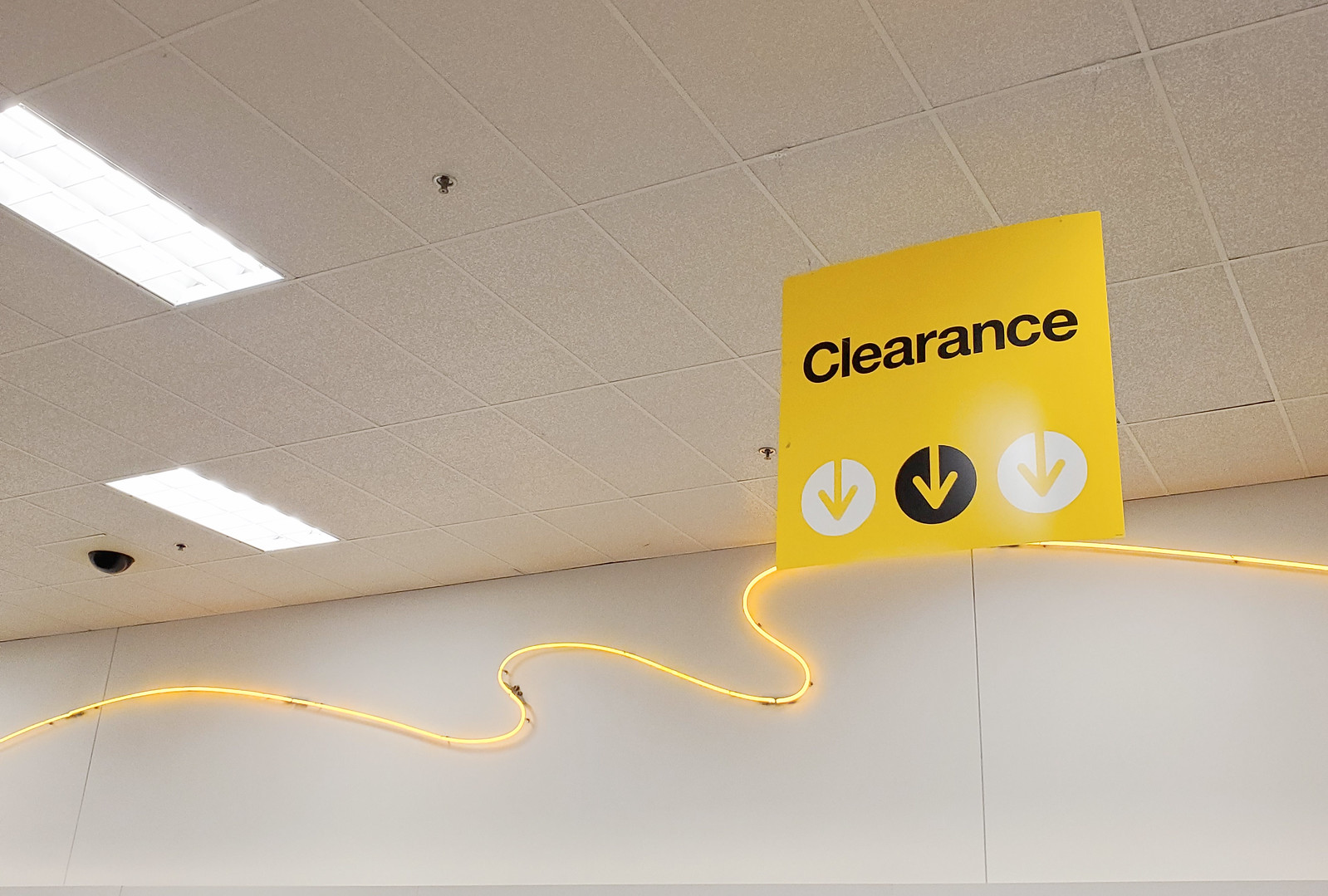A crystal-clear photograph showcases a scene featuring various elements of an indoor ceiling and wall. The ceiling is adorned with a white drop-style finish, dotted with silver fire sprinklers and fluorescent lighting fixtures. A black dome, likely housing a ceiling-mounted security camera, is also visible.

On the white wall beneath the ceiling, a wavy strip of neon light emits a golden glow. Floating above this captivating light strip, a clearance sign hangs from the ceiling. The sign has a bright yellow background with bold black font. It features three downward-pointing yellow arrows, each within a sequence of alternating black and white circles. Light reflects off one of the white circles, adding a slight gleam to its surface. Additionally, the seams of the wall are apparent, creating subtle lines that run vertically. The combination of these elements results in a detailed portrayal of the indoor environment, emphasizing both functional and decorative features.